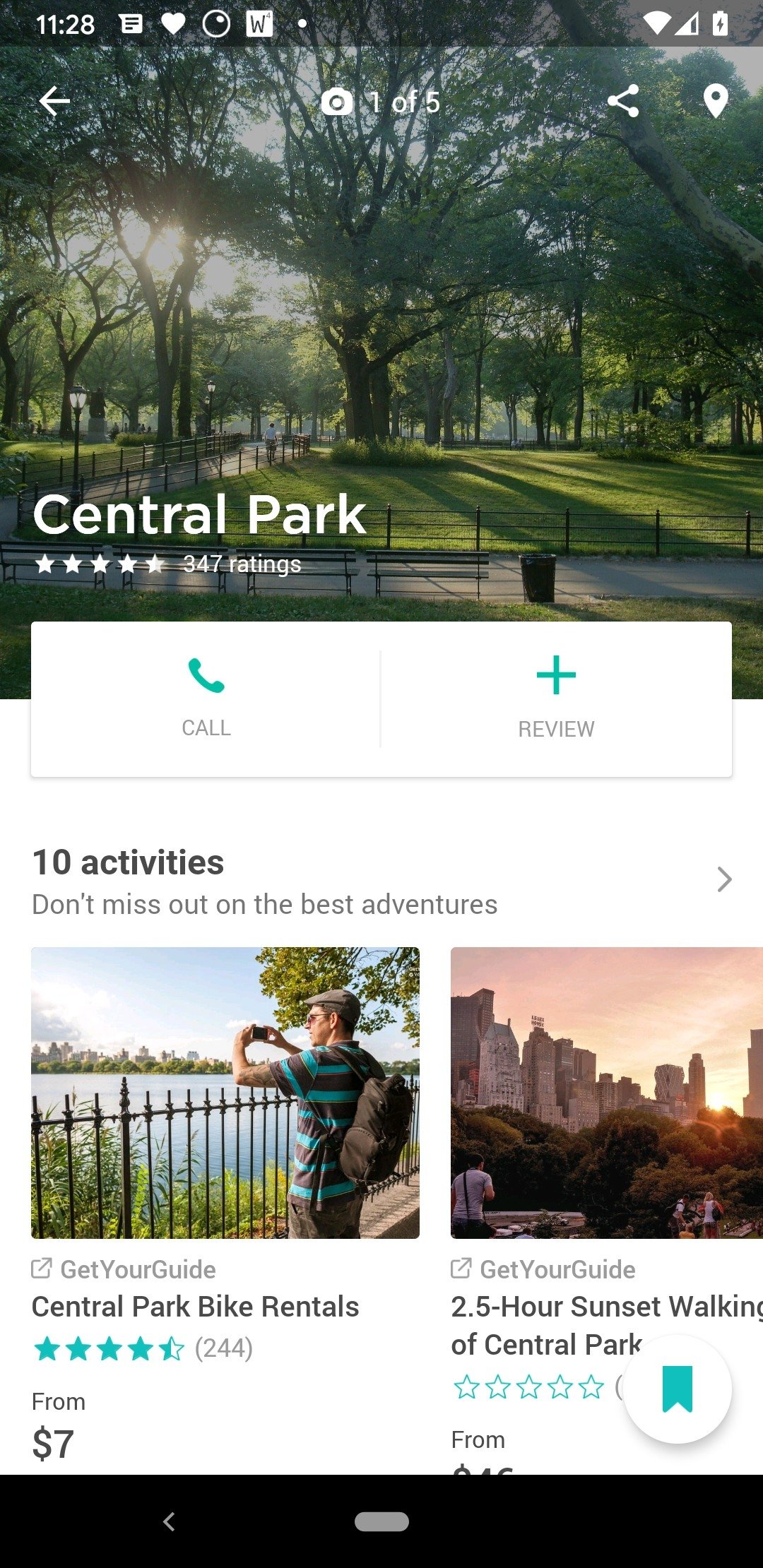**Detailed Caption:**

The central portion of the home screen for Central Park displays a picturesque scene of the park. The top third of the screen showcases the image, featuring a landscape filled with vibrant green grass and lush deciduous trees. A sidewalk cuts through the park, running from the left to the right, and diverges into the distance on the upper left, leading off into a radiant sunset. Above, the sky is a clear blue, while sunlight filters through the trees, casting a serene glow over the scene.

At the very top of the screen, a black rectangular banner spans across the width, displaying essential information in white text. On the upper left corner, the time reads "11:28," followed by icons for messages, heart, circle, and a "W." On the far right of the banner, icons show the Wi-Fi signal, signal bars, and battery life indicator.

Below the banner, a white left-pointing arrow is superimposed over the park image. At the center of the screen, there is a small camera icon with the label "1 of 5," indicating the current image in a sequence. To the far right of the camera icon, a share icon is present for easy sharing of the image.

In the lower section of the screen, the words "Central Park" are prominently displayed in white text, accompanied by a rating of five stars from 347 reviews. Below this, options for calling or reviewing are indicated by buttons. Further down, black text on a white background invites users with the message, "10 activities. Don't miss out on the best adventures."

Towards the bottom, two smaller images provide visual links to specific activities. One image is labeled "Central Park Bike Rentals," while the other advertises a "2.5-Hour Sunset Walking Tour of Central Park," enticing visitors to explore these popular options.